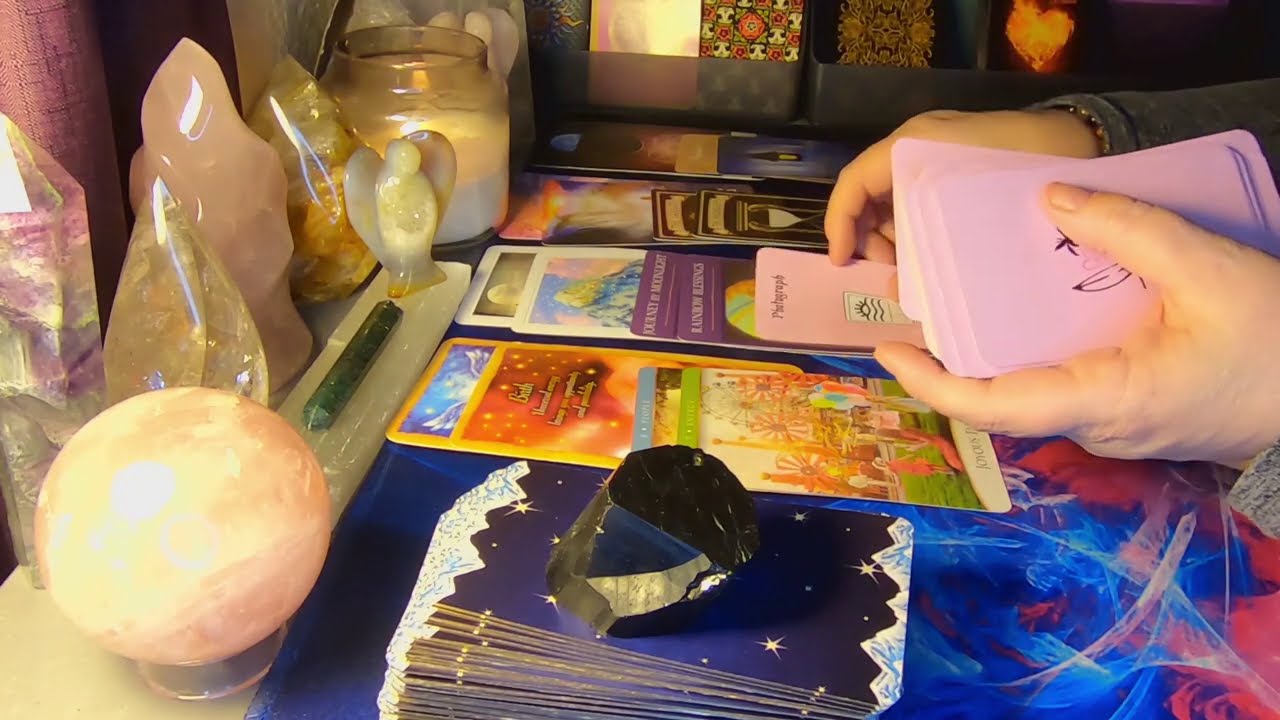The image depicts a close-up scene of a tarot card reading setup. At the forefront, a woman's hands are actively engaged with a deck of pink tarot cards; her left hand holds the deck while her right hand is in the process of pulling a single card to be laid down. She is dressed in a gray, fuzzy long-sleeved shirt and appears to be a Caucasian woman. The table surface is covered by a colorful mat with a design that includes blue, white, and neon reddish streaks, resembling a constellation pattern.

At the lower part of the image, there is a deck of blue cards with white mountain outlines, topped by a black crystal. Laid out on the table are three to four staggered rows of tarot cards. The left side of the table features various polished crystals and stones, including a spherical crystal on a glass support and a carved angel figure. Additionally, there is a large, thick jar candle burning nearby. 

In the background on the left side of the image, light filters in through a window, casting a glow on a tall, cylindrical crystal with a triangular top, giving it a purplish hue. This crystal stands before a purple curtain and is flanked by more crystals and stones, each contributing to the mystical and atmospheric setting of the tarot reading.